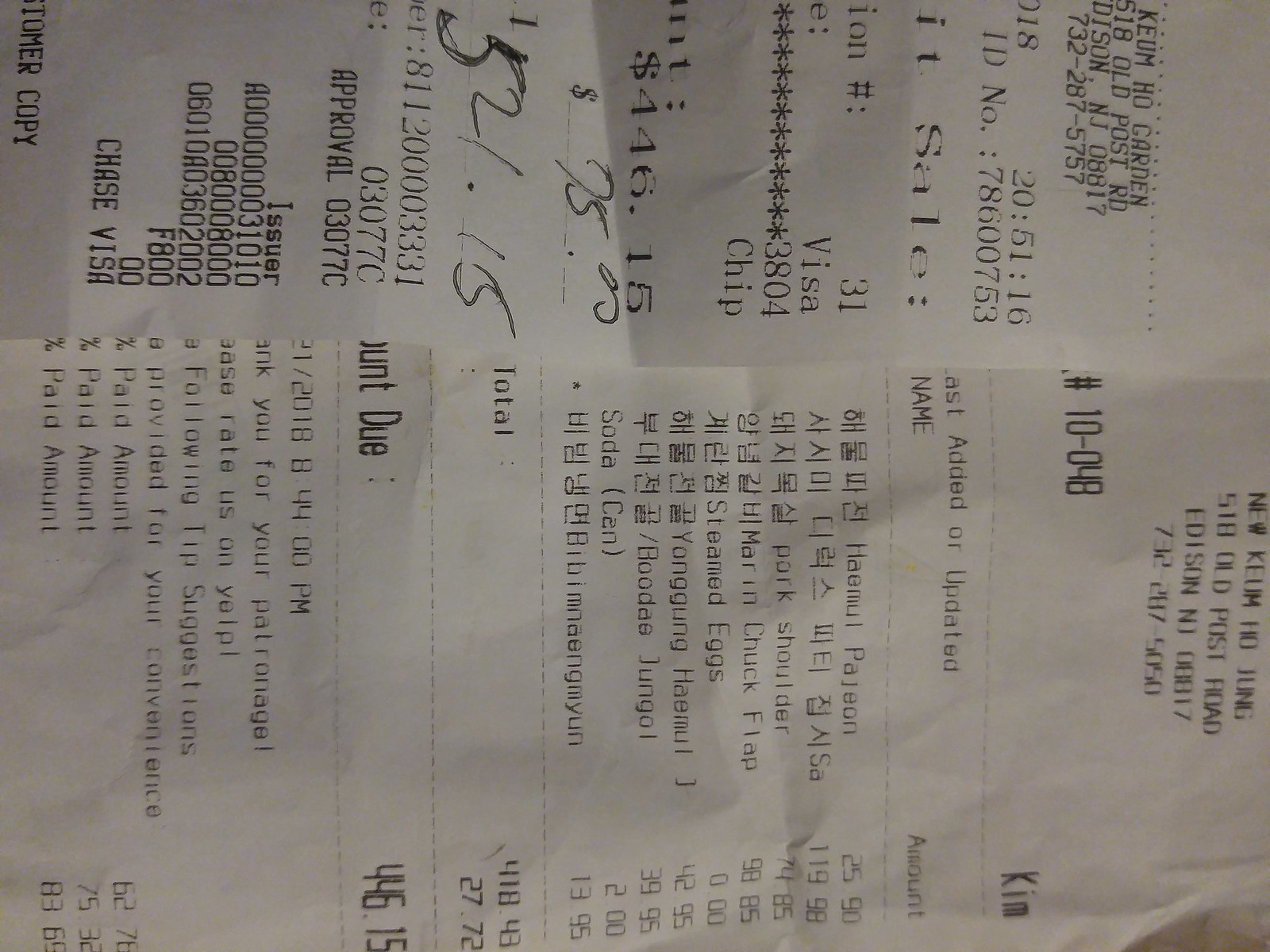This close-up photograph captures two receipts side-by-side, rotated 90 degrees to the right, making the text hard to read. The receipt on the left is partially visible, showcasing a detailed summary of a transaction. The visible portion displays handwritten numbers indicating a subtotal of $446.15 and a total amount of $521.15, with partial serial numbers, an approval code, issuer details, and payment method identified as Chase Visa. The phrase 'customer copy' is partially legible at the bottom.

The right receipt, more detailed and fully visible, belongs to "New Keum HG Jung" located at 51-8 Old Post Road, Edison, NJ 08817. The receipt lists the cashier's name as Kim, followed by itemized purchases with mixed English and Korean text. Key items include Pork Shoulder at $74.85, Marion Chuck Flap at $98.85, Steamed Eggs at $0.00, and Yong Gung Hamot at $42.95. Other items such as Soda (can) for $2 and Bibim Naengmyeon for $13.95 are also listed. The overall total is $418.43, with additional amounts adding up to $446.15, plus applicable taxes and a tip of $75.50, culminating in a final total of $521.15. Additional details include store IDs and various approval and serial codes, further detailing the transactional data.